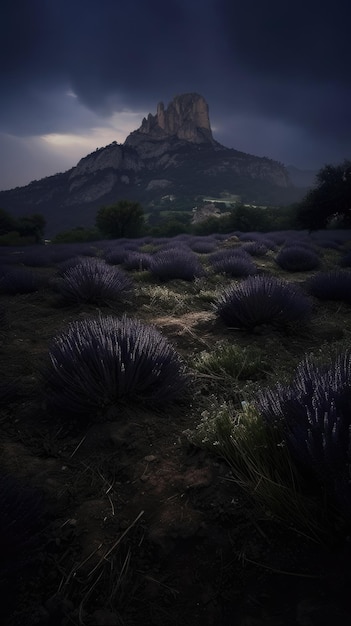This image captures a very dark, possibly stormy night scene of an outdoor landscape dominated by a rocky mountain peak. In the foreground, you can see a flat, dry expanse of land scattered with clumps of purplish, thistle-shaped bushes and plants. The ground itself presents a dark, greenish tint, adding to the overall somber mood. The mountain in the background, depicted in dark blackish-gray hues, has a lighter-colored structure atop it, possibly resembling a castle. This structure stands out against the rest of the mountain, suggesting an imposing presence. The sky is shrouded by heavy, dark clouds with just the slightest break of sunlight seeping through, accentuating the foreboding atmosphere. The scene, whether a realistic photograph or a detailed digital drawing, is rich with dark tones and textures, painting a picture of desolation and impending weather.